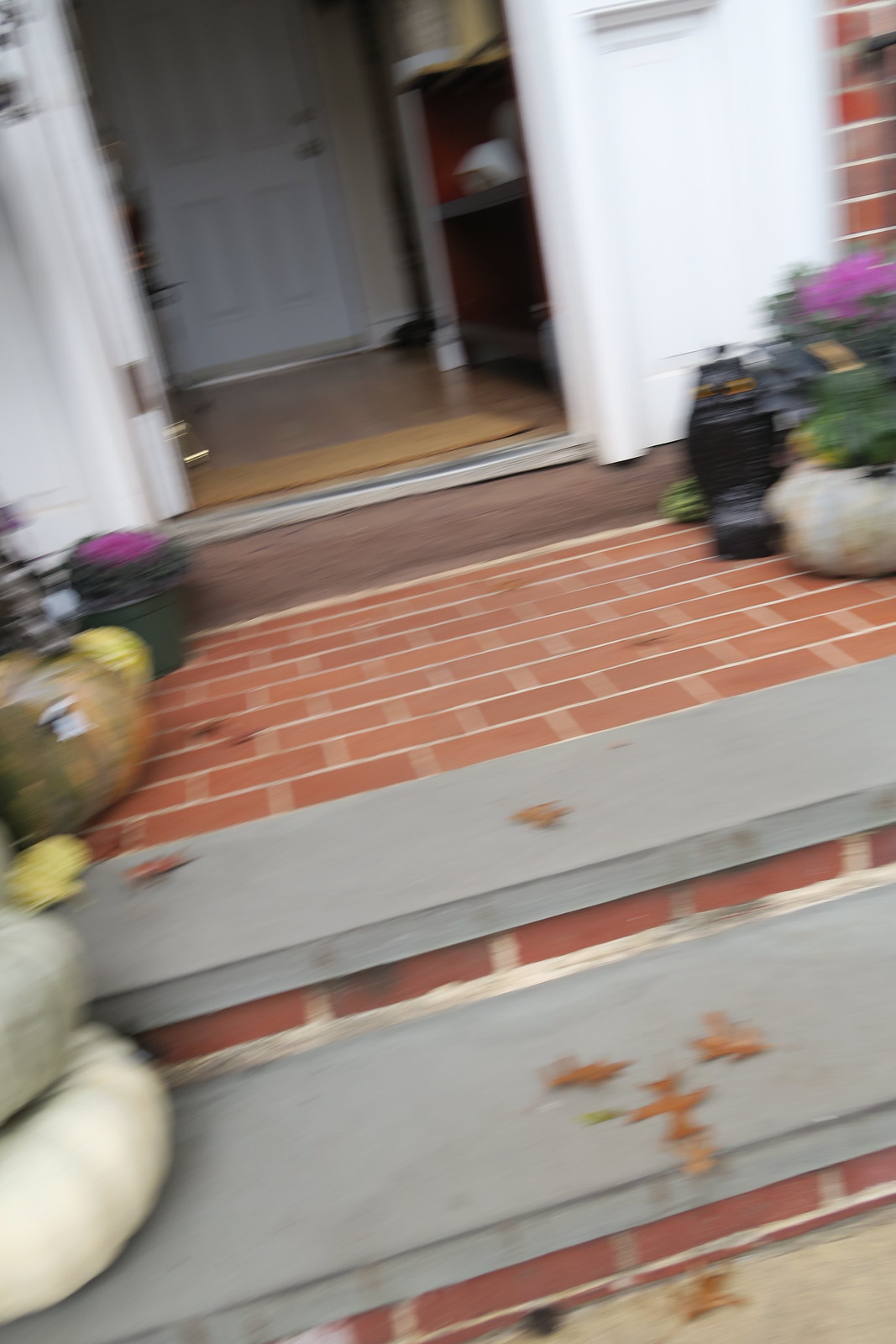The image showcases the front porch of a house featuring a red brick floor and gray concrete steps leading up to the entrance. The door is wide open, revealing a small interior room with a white door directly facing the front entrance. The porch is adorned with various seasonal decorations, including pumpkins of different colors—white, gray, orange, and yellow—placed on the left and right sides. A small black owl statue is also visible among the decorations. The scene is framed by orange leaves scattered on the steps and a brownish welcome mat at the doorway. The house's exterior is white, and inside, you can see wooden floors leading down a hallway to another white door. There are also planters with purple flowers and green leaves adding a touch of nature to the picturesque autumn setting.